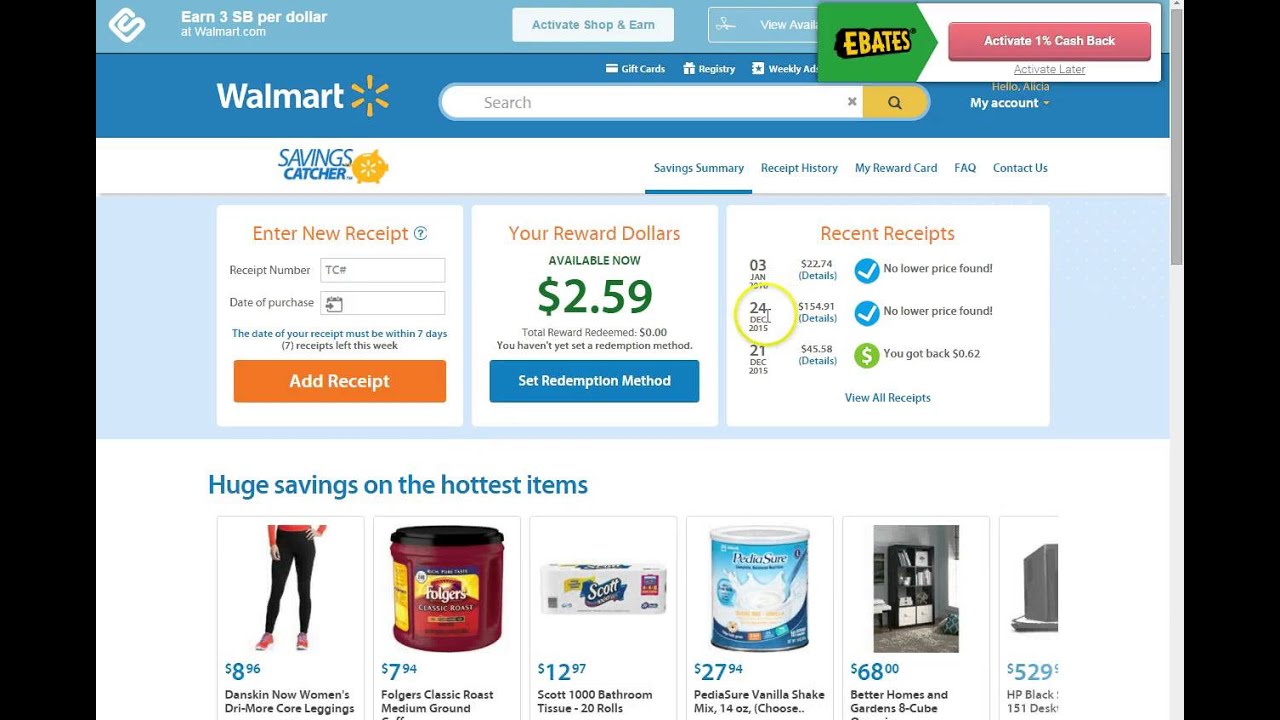The screenshot captures a page on the Walmart website, offering a detailed view from top to bottom. 

At the very top, there's a light blue promotional bar advertising an opportunity to earn 3SB per dollar spent on Walmart.com. The SB logo is situated on the left edge of this bar. Moving rightwards, the bar features two buttons: a white one labeled "Activate Shop and Earn" and a blue one labeled "View Available." A pop-up rectangle partially covering this bar advertises Ebates, offering 1% cash back with options to activate it now or later.

Directly below, the prominent signature blue Walmart bar carries the Walmart logo on the left and a central search bar with options for gift cards, registry, and weekly ads positioned above it. On the right side of this bar, a yellow-font text greets, "Hello, Alicia," next to a white-font dropdown menu for "My Account."

Beneath this, a white navigation bar labeled "Savings Catcher" lets users switch between tabs such as Saving Summary, Receipt History, Reward Card, FAQ, and Contact Us. The "Saving Summary" tab is highlighted, indicating the active view.

The main content area features three distinct sections. On the left, a box allows users to enter new receipt details based on the number and purchase date. The central box displays reward dollars available, prominently showing "$2.59" in green font. The right box lists recent receipts, detailing the date, total price, and any found savings or reimbursements. 

At the bottom, a blue-font message promotes "Huge Savings on the Hottest Items" accompanied by images and prices of six featured products: leggings, Folgers coffee, toilet paper, baby formula, and shelving units.